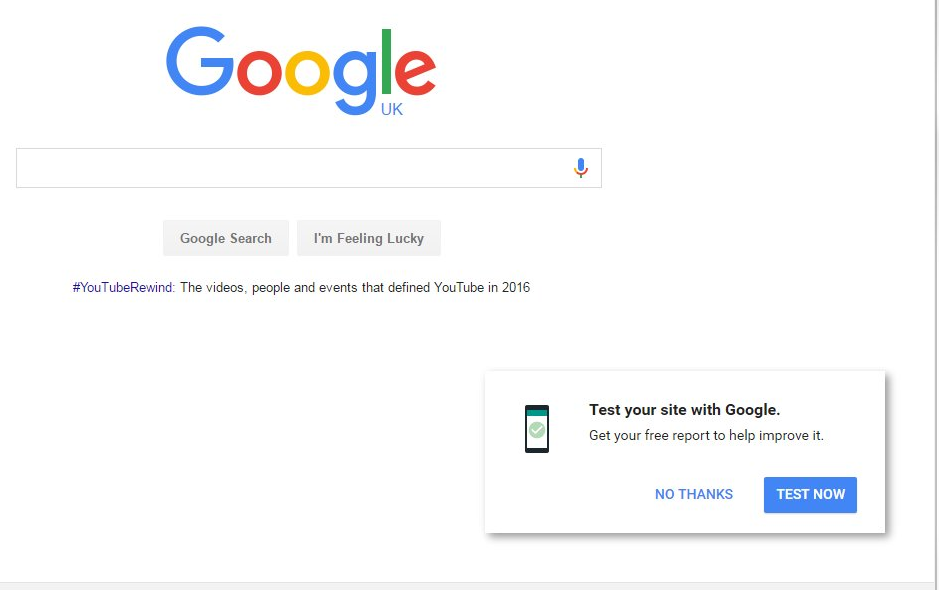Screenshot of Google UK Homepage: The image is a partial screenshot of the Google UK homepage. The iconic Google logo is situated on the left side rather than being centered. Directly below the logo is a search box which includes a small microphone icon to the right. To the left of the search box, "Google Search" and "I'm Feeling Lucky" buttons are visible.

Beneath these buttons is a gray hashtag "#YouTubeRewind," followed by a description highlighting the videos, people, and events that defined YouTube.

At the bottom right corner, the image shows a small, white text rectangle with a shadow, which contains a prompt: "Test your site with Google. Get your free report to help improve it." On the left of this prompt is an icon of a mobile phone displaying a black and green bar at the top and a green checkbox. The prompt box also includes two buttons: "No thanks" in blue text on the left and "Test Now" in white text with a blue background on the right. This partial view of the page does not show the full layout and edges, suggesting the screenshot is cropped.